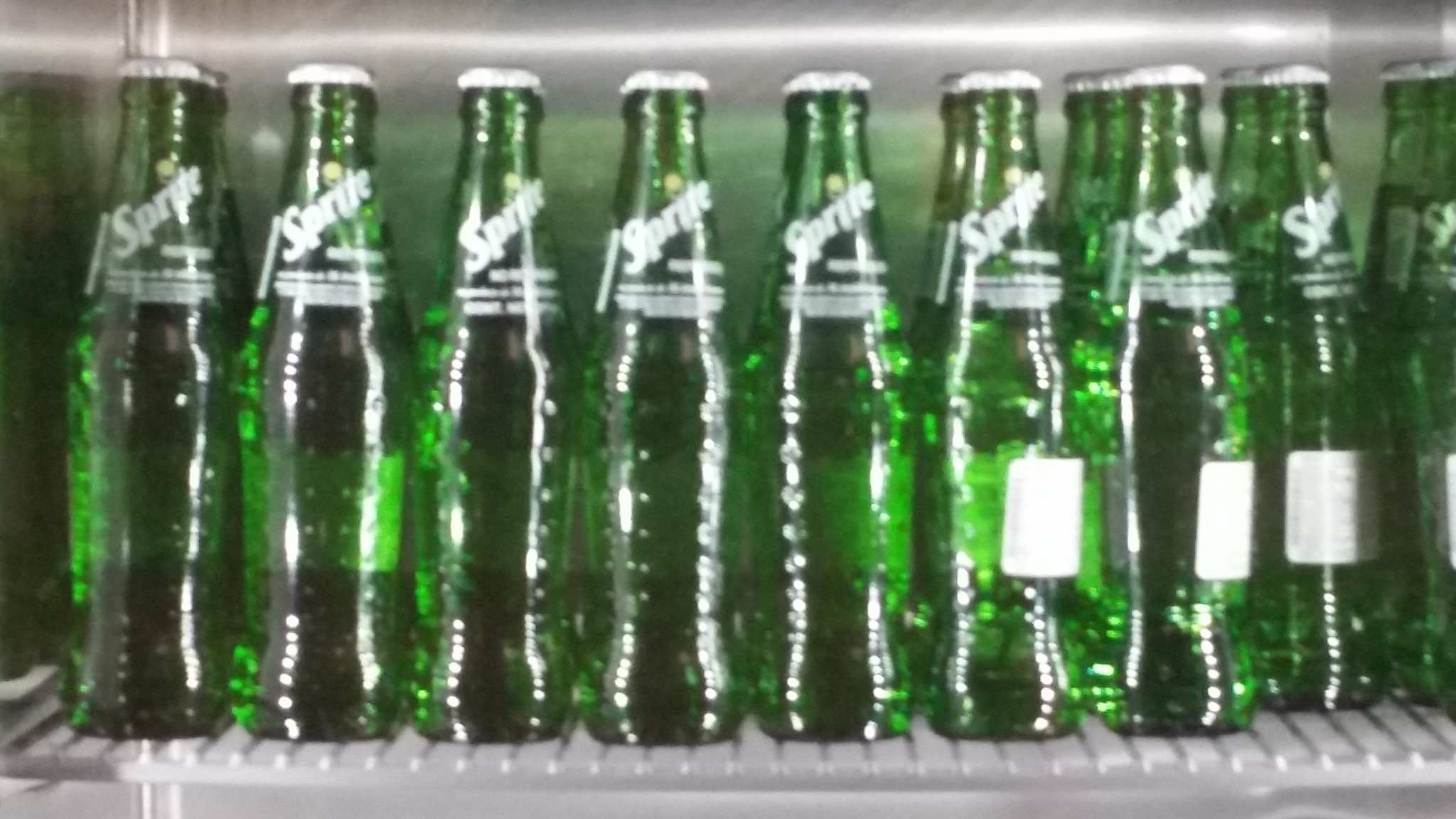This somewhat blurry photograph captures a nostalgic view of a cooler filled with Sprite bottles, reminiscent of the late 80s. Inside a steel refrigerator with reflective metal walls and a silver wire rack shelf, there are approximately nine green, textured glass bottles arranged in a neat row. Each bottle features a white Sprite logo, displayed diagonally from left to right near the neck, and crowned with a classic silver metal cap that requires a bottle opener. Some bottles have white square labels visible towards the right side of the image. The bottles’ shoulders are wider, tapering down to a narrower neck and rounded bottom, adorned with dotted texturing meant for better grip. Though slightly obscured by the photo's angle and lack of focus, the arrangement shows multiple rows of bottles behind the front line, emphasizing the stocked appearance of this vintage scene.